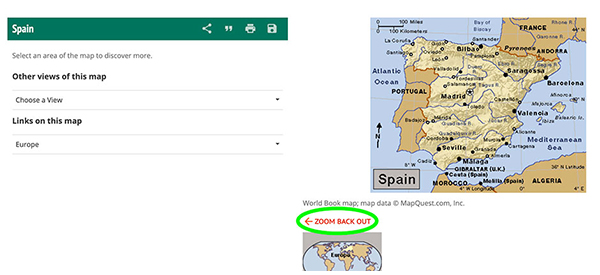This image captures a screenshot from a tablet device, displaying an old MapQuest interface focused on Spain. The dimensions appear suited for a tablet, being too large for mobile and too small for desktop use. 

The main feature is a long, white rectangular map. In the top-left corner, a green bar prominently displays the word "Spain" in white text. Adjacent to this, several small icons are visible including a share icon, a quotation mark-like icon, a printer icon, and a potential file download option, though their diminutive size makes identification challenging.

The interface instructs the user to "select an area of the map to discover more." Located to the right is the map itself, which shows Spain along with its neighboring countries—France, Portugal, and Algeria. Notable Spanish cities such as Madrid are also visible.

Beneath the map, a prompt reads "Other views of this map," suggesting that there are additional perspectives available through a drop-down menu for Europe and possibly other regions.

Towards the bottom of the interface, there is a label: "World Book Map" and a source citation, "mapdata @ mapquest.com." Highlighted in green within an oval, another red-highlighted option advises the user to "zoom back out" for a global view, instead of just Spain.

Overall, this screenshot encapsulates an interactive map experience from an older version of MapQuest, integrating options for detailed exploration and view customization.